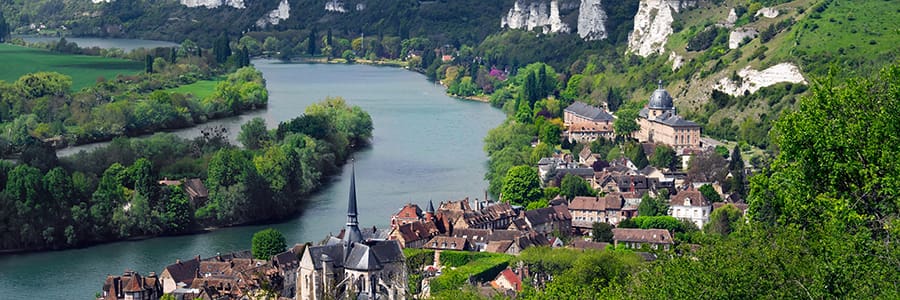The image is a color photograph taken from a high vantage point, likely a hillside or via a drone. It showcases a picturesque view of the Seine River in France, elegantly snaking through the landscape from the bottom left corner towards the center, then curving back up to the top left. The river, a dark greenish-blue, is flanked by lush green trees along its banks and peppered with small inlets.

On the left side, a prominent church with a dark blue spire stands out among several other towers. Next to the church, red tile-roofed buildings extend along the riverbank, following its natural curve. This village comprises houses, possible apartment buildings, and businesses, forming a vibrant community. Towards the lower right corner of the image, green trees are visible, enhancing the lushness of the scene.

In the upper right portion, the incline of the land becomes steeper, marked by white rock outcroppings and sheer cliffs. Below these cliffs, there is a domed structure among the greenery. The landscape continues with grassy inclines and scattered trees, blending seamlessly with the built environment. Overall, the composition, steeped in photographic realism, captures the serene beauty of the Seine River and its charming riverside village.